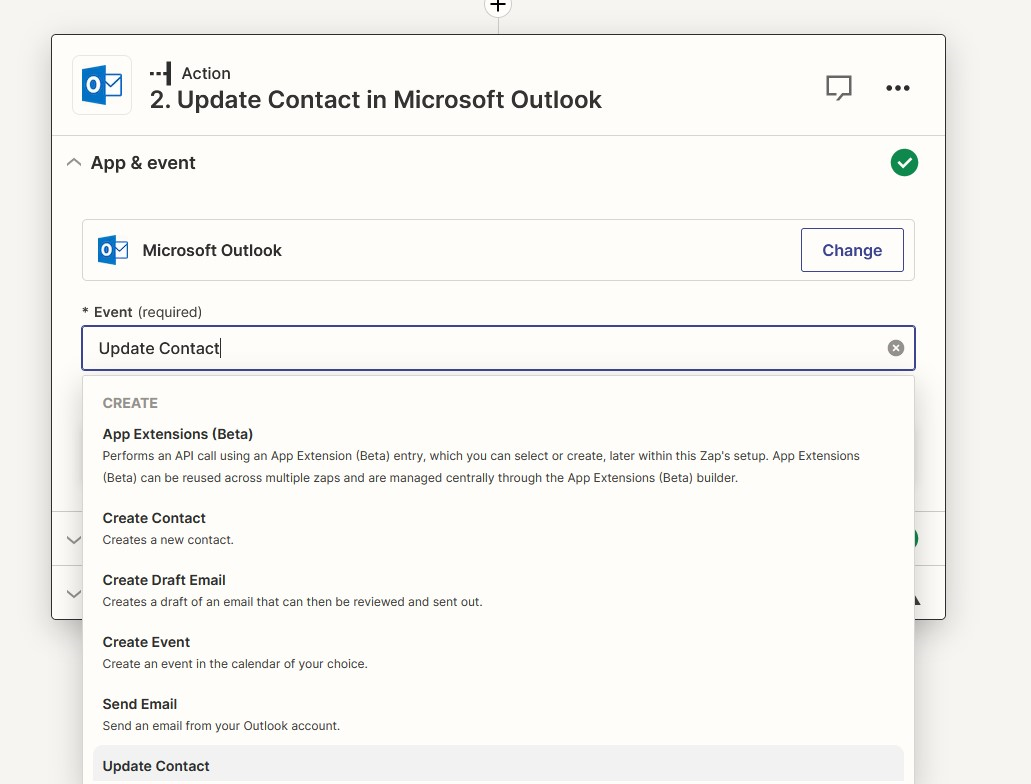**Caption:**

A detailed screenshot of the process for updating a contact in Microsoft Outlook. In the upper left-hand corner, the familiar Microsoft Outlook icon is visible, featuring an envelope and a square box with a zero inside. In the top strip, which takes up about 10% of the page, there are various icons including a note, three dots, and an up arrow. The interface also shows "app and event" options, accompanied by a green check mark, indicating a successful action. 

Directly below the Microsoft Outlook header, the "Update Contact" link is highlighted. An input box for updating contact details is present, suggesting an active search or input function. The screenshot details various options such as ‘Create,’ ‘App Extensions Beta,’ which performs API calls using the App Extensions Beta entry, and allows you to either select or create extensions later, managed centrally through the app extensions beta builder.

Additional options include:
- **Create Contact:** To create a new contact.
- **Create Draft Email:** To draft an email that can be reviewed and sent out.
- **Create Event:** To create an event in a calendar of your choice.
- **Send Email:** To send an email from your Outlook account.

The entire interface is set against a clean white background, ensuring clarity and ease of navigation for the user.